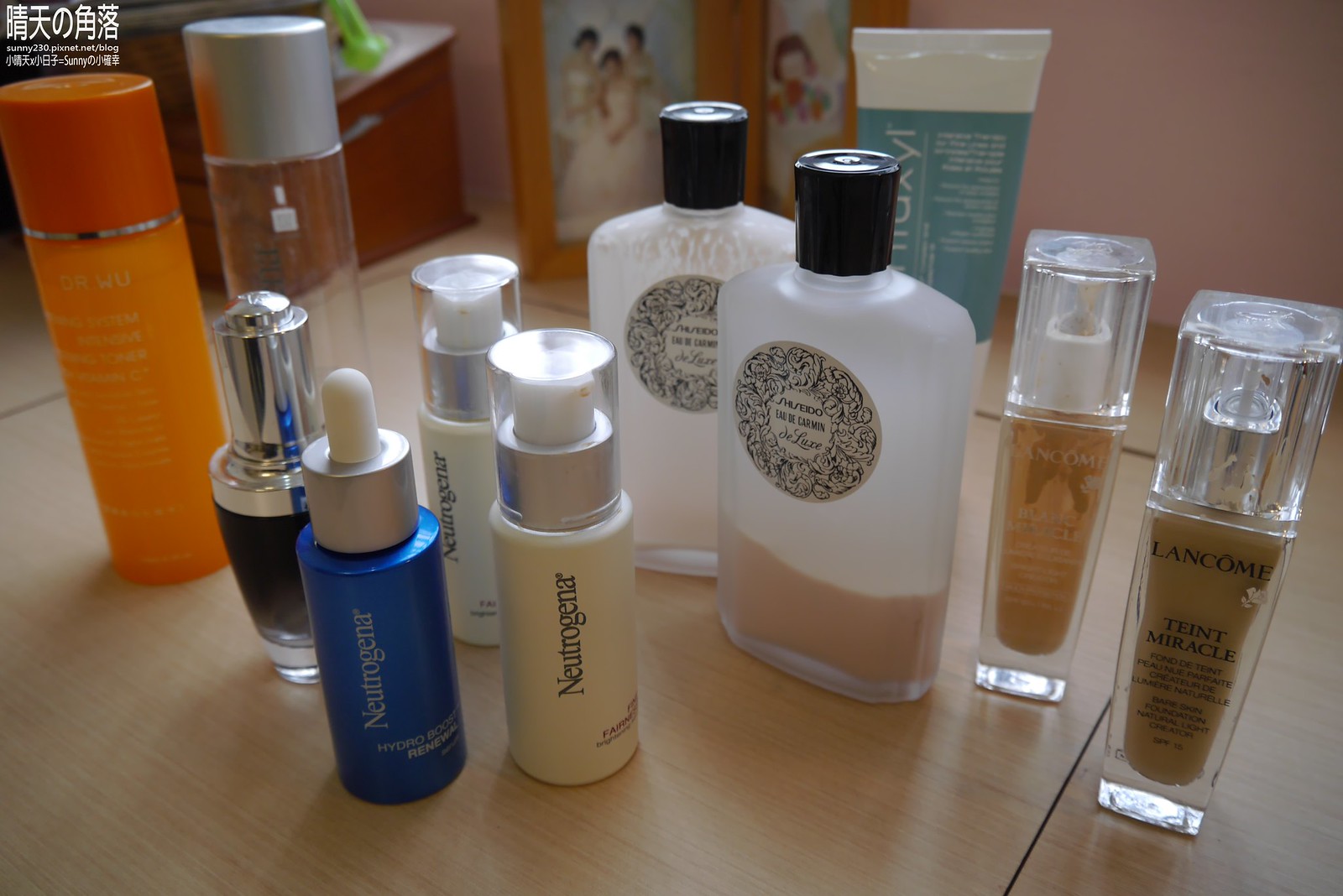In the photograph, a neatly arranged collection of cosmetic bottles is showcased on a pale wood-finished corner shelf, situated in either a bathroom or a bedroom. The backdrop is a soft pink wall, enhancing the serene ambiance of the setting. 

From left to right, the items on the shelf include:

1. A series of Chinese characters printed in white against a slightly blurred background.
2. A double photo frame in the center, displaying a wedding photo on the left featuring three dark-haired women, with the bride prominently positioned at the front, and another wedding photo partially visible on the right.

The following cosmetic items are precisely organized across the surface:

1. A tall, slender orange bottle.
2. Beside it, a fair bottle with a metallic gray cap.
3. A shorter glass bottle with a black label and a shiny chrome cap situated just below.
4. In the foreground, two vertically labeled Neutrogena bottles – one dark blue with white lettering and another off-white or creamy with black lettering, both capped in white.
5. Directly behind these, another Neutrogena bottle.
6. Two similar-looking, broad yet slender bottles featuring circular cream and black labels, partially readable as "OD something-or-other deluxe."
7. On the far right, two Lancome bottles with clear bodies and clear caps.
8. Finally, a white and pale blue tube of an unidentified product sits at the back line.

The entire scene exudes a sense of meticulous organization and cleanliness.